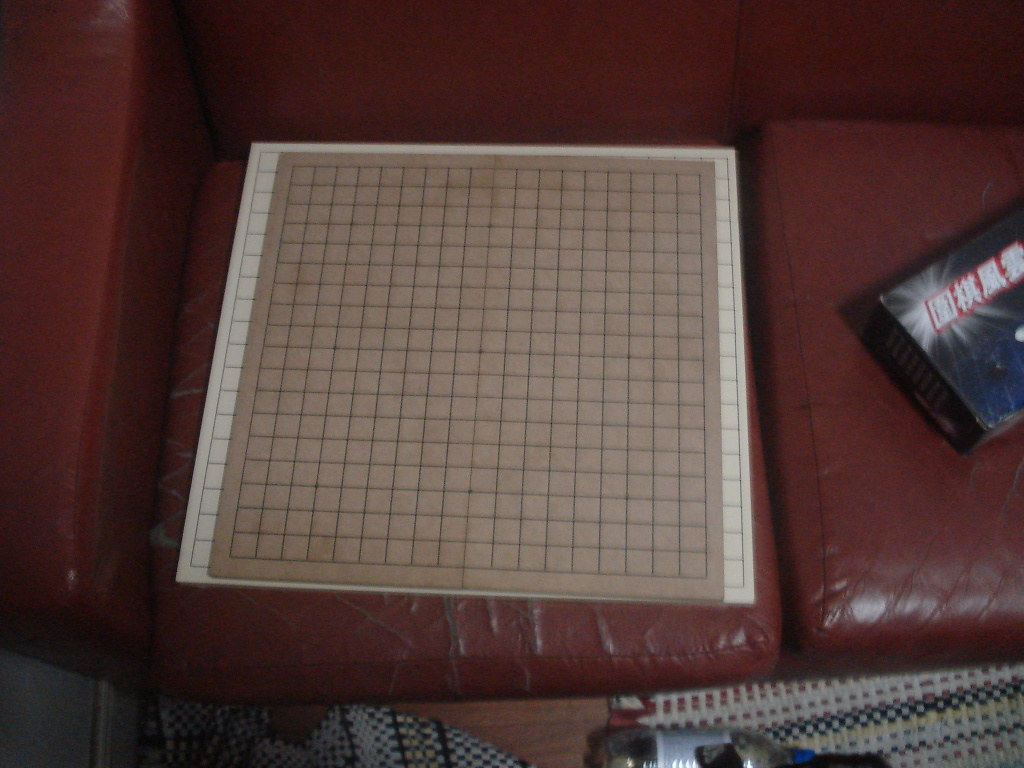This image is a top-down view of a distressed, red-brown faux leather couch, focusing on one worn cushion and part of an armrest. Centrally placed on the cushion is a game board, which could potentially be a Go board, suggested by the grid of numerous black-lined squares, bordered in white. In the background, a slender, partially visible box with Japanese or Chinese writing implies an Asian origin of the game board. Below the couch, parts of two rugs with similar black, yellow, and white patterns are discernible. Additionally, a bottle is visible on the floor, hinting at a lived-in environment. The intricate details in the scene suggest a blend of play and casual setting.